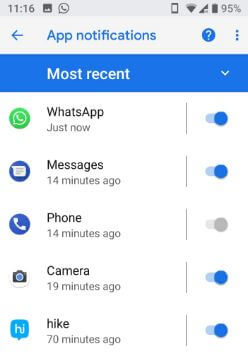**Detailed Caption:**

The image displays a close-up of a cell phone screen with intricate details. 

At the top-left corner, there is the time "11:16" in white font. To the right of the time, there is a small picture icon followed by what appears to be a message indicator. The phone is set to vibrate or silent mode, as indicated by the relevant icon next to the message indicator. Further right, the screen shows the signal strength bars and the WiFi or data signal icon. The battery status is prominently displayed at "95%".

Below these indicators is a section featuring a left arrow icon, several app notifications, a circle icon with a question mark, and three vertical dots, all of which are displayed in blue font.

The top portion of the screen displays a blue strip with the text "Most Recent" in white, accompanied by a downward-facing arrow on the right.

Beneath the blue strip, there is a list of recent app activities:
- "WhatsApp: Just now," which is toggled on (green slider).
- "Messages: 14 minutes ago," also toggled on (green slider).
- "Phone: 14 minutes ago," toggled off (grey slider).
- "Camera: 19 minutes ago," toggled on (green slider).
- "Hike: 70 minutes ago," toggled on (green slider).

The colors used in the interface are primarily grey, black, white, blue, and green, with various shades of each color. The image appears to be significantly enlarged, filling the entire screen of a large tablet, causing pixelation and blur due to the increased size and resolution limits. This enlargement emphasizes the screen's details but may slightly distort the clarity.